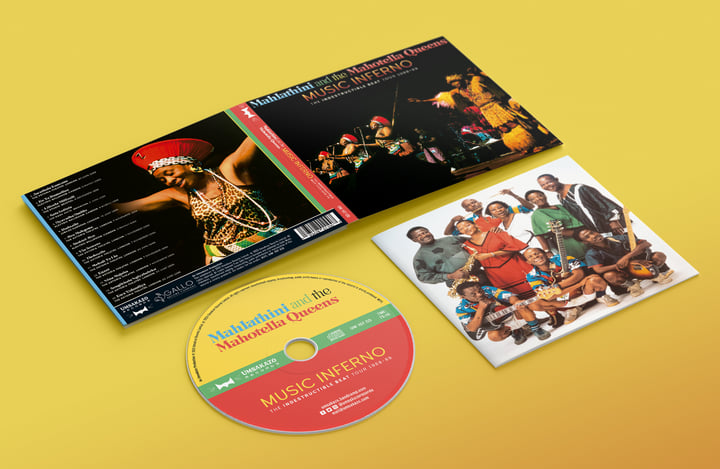In the image, there is an open album case laid flat, revealing both its interior and contents. On the left side, the back cover features a woman in a red hat with white trim, adorned with long white beads and wearing a sleeveless jaguar skin blouse. She appears to be dancing. Above her is the song list against a brownish-yellow background. The right side displays the album's front cover, showing a band in traditional African attire, performing music on a stage. Below this cover, the title "Malathani and the Mahotella Queens, Music Inferno" is prominently visible. The CD, positioned diagonally, is striking with its yellow and red color palette, accented by a green strip. The CD itself clearly states "Music Inferno" in yellow lettering, and the band's name is colorfully rendered with "Malathion" in blue, "And" in green, "The" in black, and "Mahotella Queens" in red. Beside the CD, there is a picture of several band members, with three holding guitars, contributing to the vibrant scene.